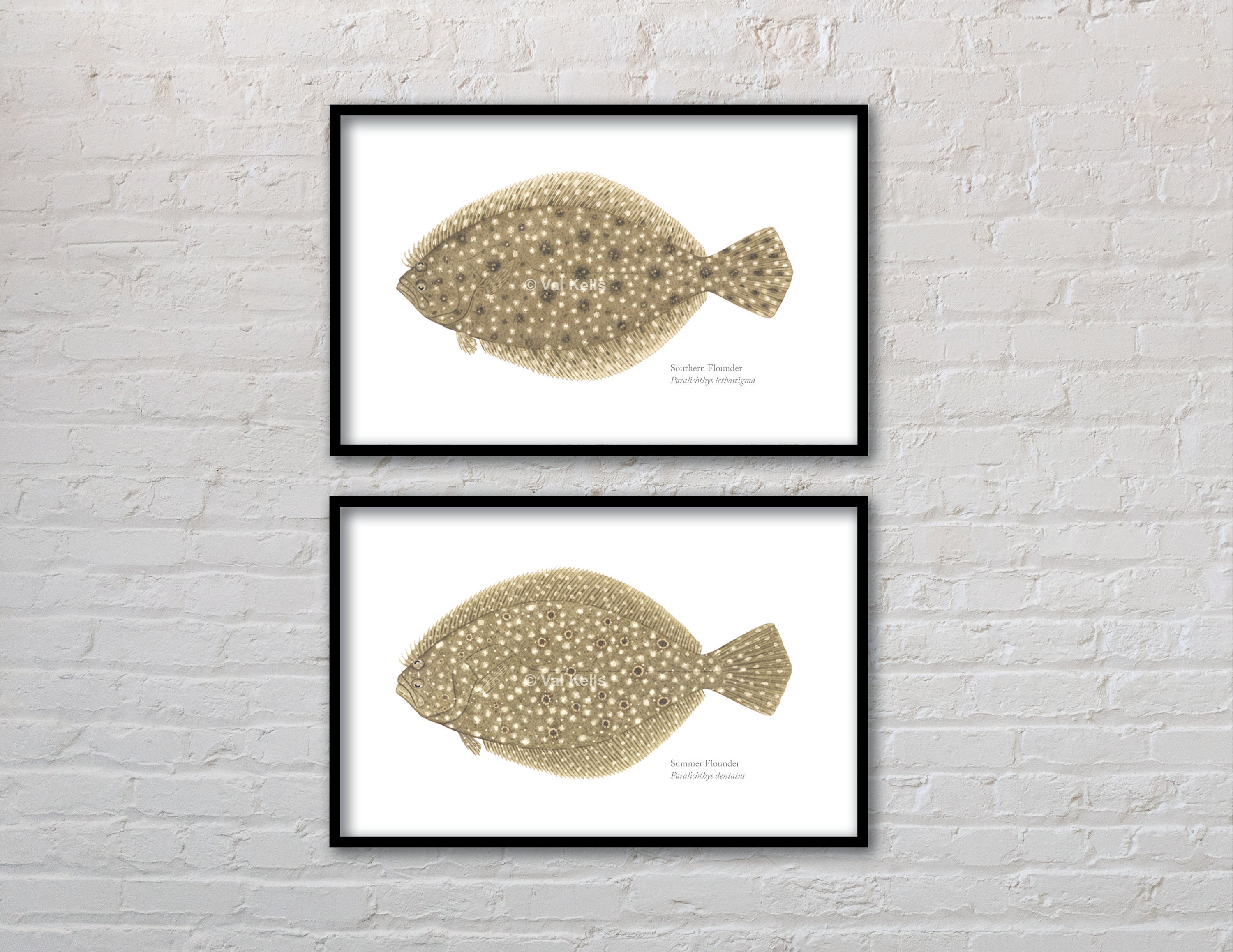This photograph depicts two rectangular art prints of flounder fish, displayed vertically on a white-painted brick wall with a small gap between them, approximately the height of one brick. Each print is enclosed in a thin black frame. The top print features the Southern Flounder, labeled with its common name and the scientific name "Paralichthys lethostigma" in small, black text. This fish is wide-bodied, with large, thin fins adorned with numerous black and white dots. The image includes a white copyright watermark reading "Val Chemis" across the center, again spelled "V-A-L-K-E-M-S."

The bottom print shows a Summer Flounder, similarly labeled with its common name and the scientific name "Paralichthys dentatus." Unlike the top fish, the Summer Flounder has fewer black dots, more prominent white dots, and darker scales; its fins also feature black circles with white outlines. Both fish drawings are set against a white background, highlighting their detailed, dot-patterned bodies.

Overall, the prints emphasize intricate fish illustrations with subtle variations in dot patterns and colorations, graphically capturing the characteristics of each species.